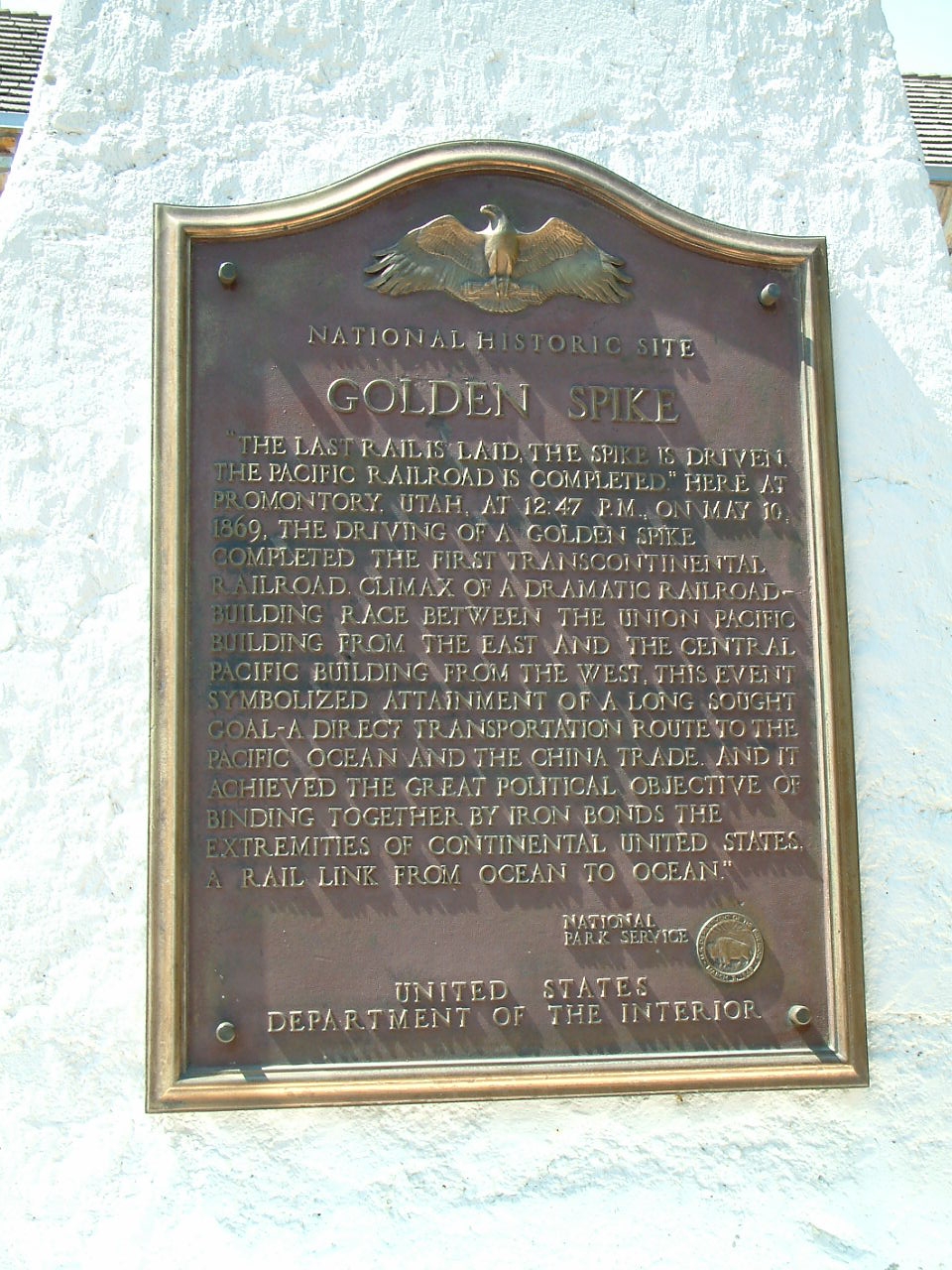The image shows a rectangular bronze plaque set against an outdoor white stone wall. The plaque features a gold-edged border with a prominent beveled top, and a gold eagle with outstretched wings is centered at the top of the plaque. Beneath the eagle, in embossed metallic letters, it reads "National Historic Site, Golden Spike." The plaque commemorates the completion of the first transcontinental railroad at Promontory, Utah. It details that on May 10, 1869, at 12:47 PM, the driving of a golden spike marked the union of the Union Pacific building from the East and the Central Pacific building from the West, symbolizing the attainment of a direct transportation route to the Pacific Ocean and China trade. This event is celebrated as a significant political accomplishment in binding together the continental United States with an iron rail link from ocean to ocean. At the bottom right corner of the plaque is the seal of the National Park Service, featuring a buffalo, alongside the text "United States Department of the Interior."